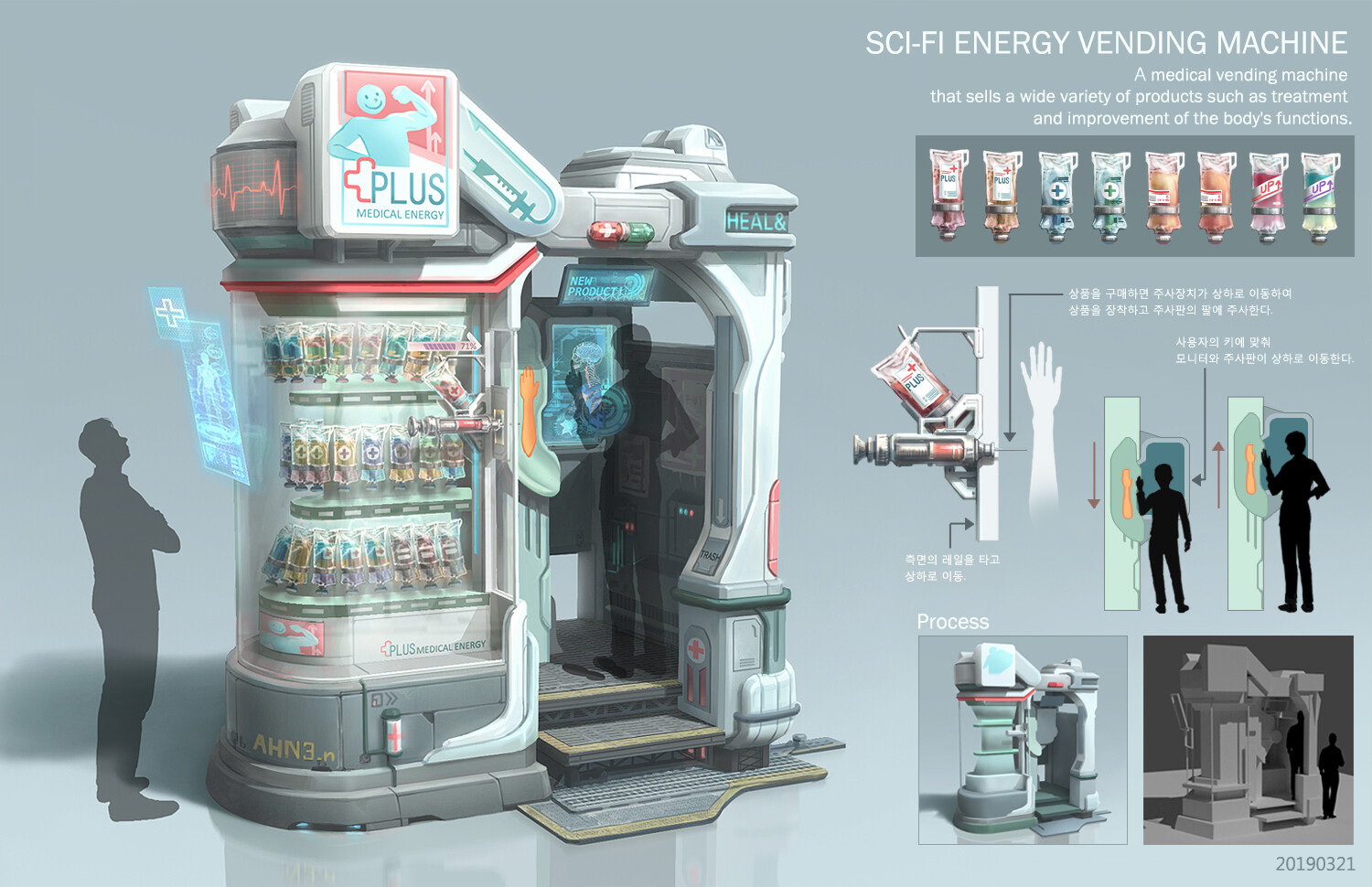This illustration is an advertisement for the "Sci-Fi Energy Vending Machine," a futuristic medical vending machine designed to dispense a wide variety of products aimed at treatment and improvement of bodily functions. The top right of the image prominently displays the title "Sci-Fi Energy Vending Machine," followed by a description emphasizing its medical purpose. The vending machine, referred to as "CrossPlus," has a curve-shaped design and features a monitor on the inside where users select their desired products via touchscreen.

On the left side of the image, the vending machine is depicted in detail: it has a sleek, gray base and a transparent glass display showcasing various products, including colorful liquid-filled pouches resembling blood pouches. These pouches come in different colors such as orange, green, and blue, suggesting different types of medical treatments. Above the machine, a "Plus Medical Energy" sign is accompanied by a heart rate monitor graphic and the word "HEAL" in blue text.

To the right of the machine, inset illustrations provide additional details, including diagrams in a foreign language, possibly Korean or Chinese, outlining the machine’s operation and the types of products available. One diagram depicts a package with a needle, indicating that these products might be injectable. Silhouetted figures in black are seen interacting with the machine, suggesting its user-friendly design.

Overall, the illustration combines elements of sci-fi aesthetics and medical technology, presenting a comprehensive and detailed visual description of the Sci-Fi Energy Vending Machine’s features and functions.